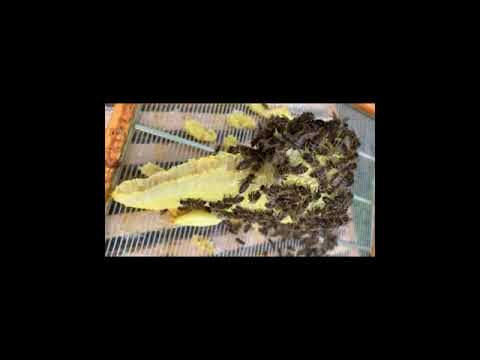The photograph, taken from above and framed by a thick black border that occupies around 60% of the overall image, showcases a scene centered around a rectangular silver grate positioned on a wooden surface. Despite the small size of the photograph within its border, which makes details somewhat blurry and difficult to discern, certain elements stand out. At the center of the grate lies a long yellow object, potentially a honeycomb, fish, or even a piece of corn or romaine lettuce. This yellow object is heavily swarmed by numerous brownish-black insects, most likely bees, suggesting a beehive scenario. The bees are densely congregated over the object, which appears to be the focal point of their activity. The setting seems to be outdoors, given the wooden edges and natural context, possibly indicating that the tray beneath the grate is used by professional beekeepers. The intricate details and busy scene, though cryptic, paint a picture of nature and industriousness.